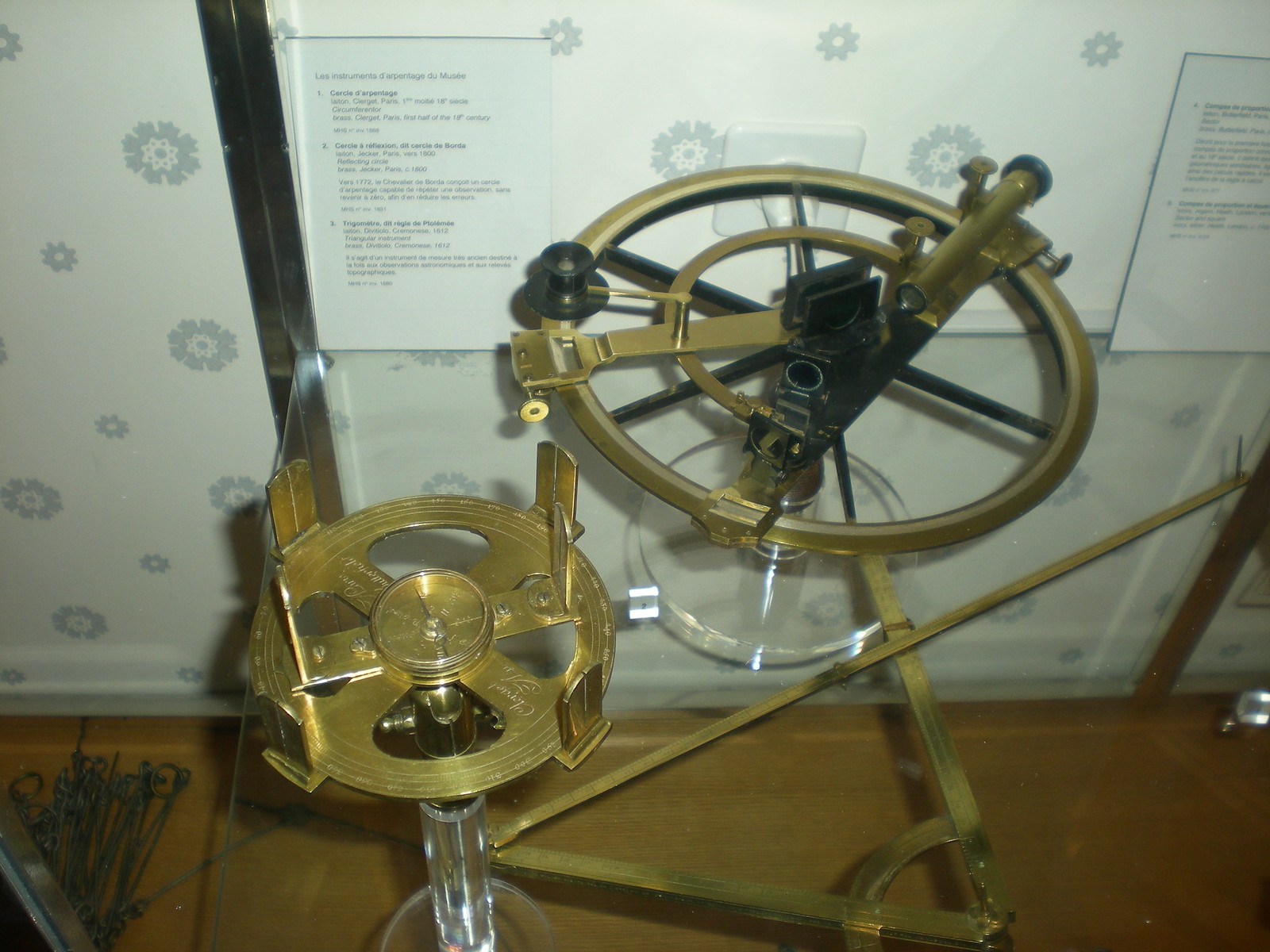This image depicts a museum display featuring two interconnected circular devices, crafted from gold or brass, which are mounted on a glass stand. The larger wheel is accompanied by a smaller one, both forming a notable feature of some intricate machinery. Behind the wheels, set against a white wall adorned with subtle grey floral patterns, are several informational sheets, though the text on these sheets is not legible. To the left of the wheels, a cluster of metal wires with small hoops at their ends is visible. The display is positioned on a wooden floor, with a brown table visible beneath the apparatus.